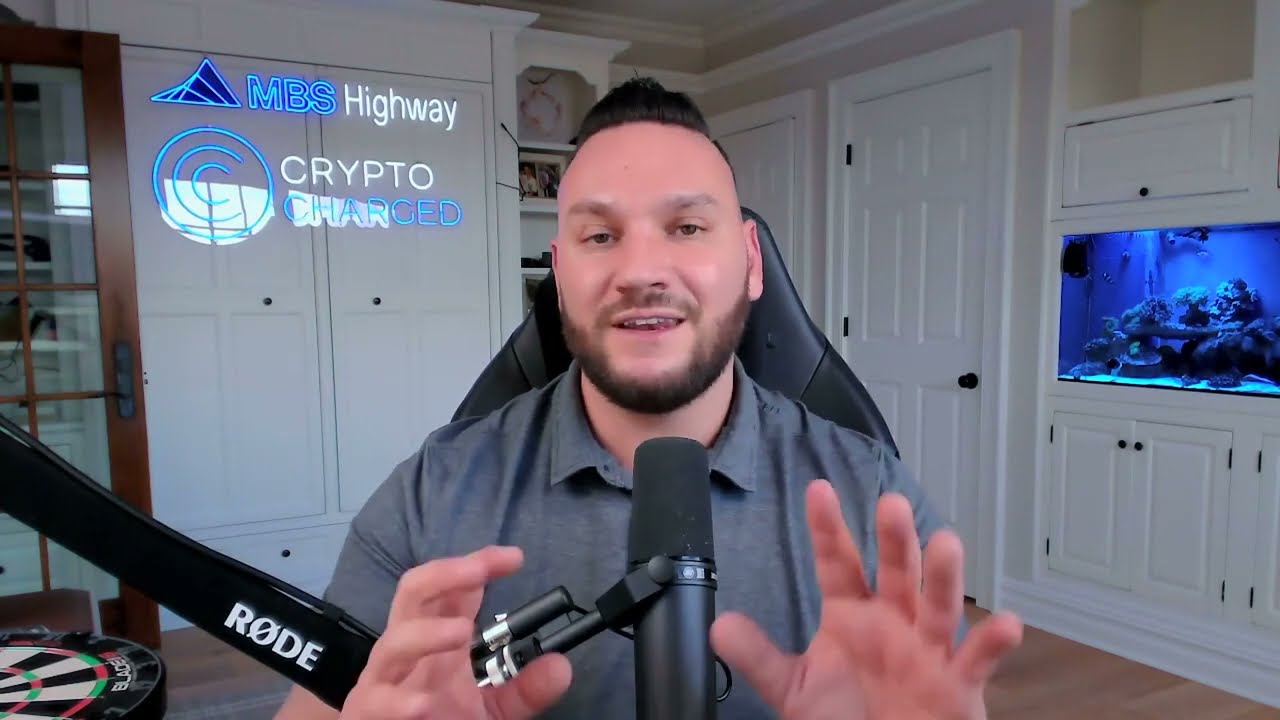The image depicts a Caucasian male, likely in his 30s or early 40s, broadcasting from his home office. He has short, slicked-back brown hair with the sides of his head shaved, complemented by a closely trimmed full beard and mustache. He is seated in a high-backed black gaming chair, wearing a dark gray short-sleeved button-up collared shirt. The man is actively speaking, with his hands raised and fingers spread as if emphasizing his points. A shotgun microphone on a boom stand is directed towards his mouth from above. The webcam, positioned atop his computer, records him in what appears to be a dining room converted into a home office, evidenced by the fish tank installed in the wall and an abundance of white cabinets, closets, and shelves. Blue-lit text in the upper left corner reads "MBS highway crypto charged," adding a professional or thematic element to the scene. The ambient daylight floods the room, clearly indicating that the recording is taking place during the day.